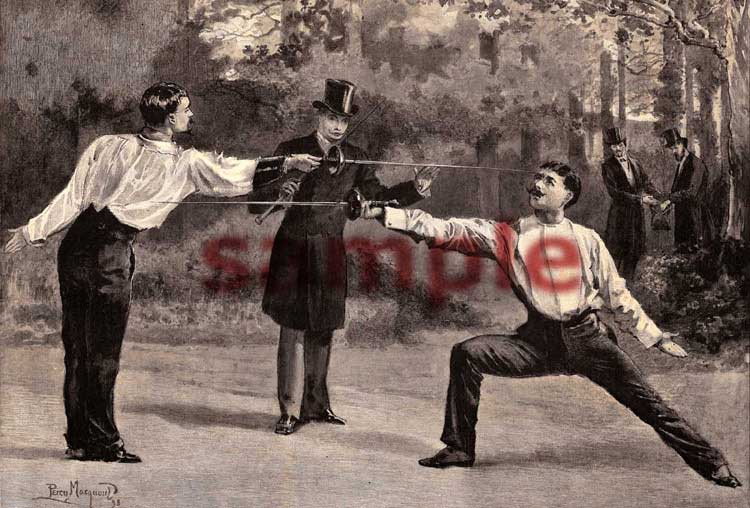In a detailed and vintage monochrome drawing, the central scene captures two men engaged in a sword fight, both clad in black pants and long-sleeve white shirts. One man, observed from behind on the left, is extending his right arm with a thin, fencing-like sword towards his opponent. His left arm hangs by his side. The other man, positioned on the right and seen from the front, has one knee bent as he thrusts his similar sword towards the first man. Between them stands a mediator, possibly a referee, dressed in a long black coat and top hat, holding a stick to oversee the duel. The background features a blurred landscape of trees and bushes. Additionally, in the distance towards the right, two smaller figures, also in black coats and top hats, observe the scene. Subtle text is visible at the bottom left and a red "sample" watermark overlays the center of the image.